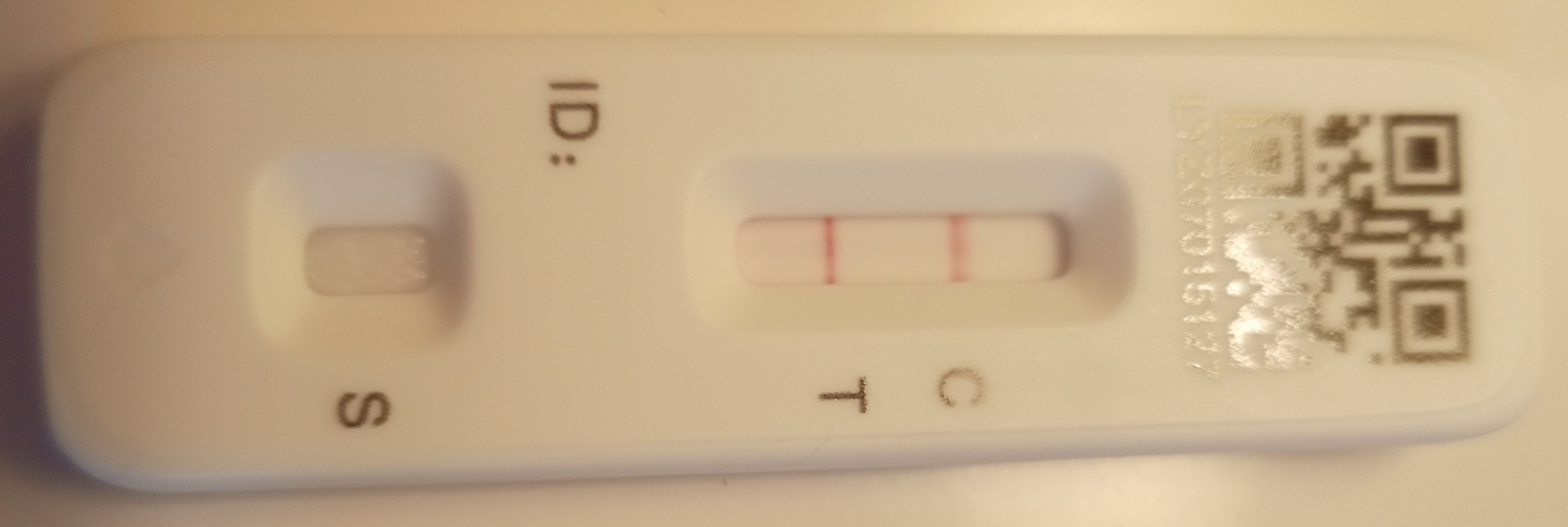This photograph captures a blurry image of a COVID-19 rapid test on a white matte background. Due to unclear lighting, the background could be a counter, a wall, a floor, or even a piece of paper. The test device itself is a slim, white tablet-like structure. At the top, there's a QR code, and below it, partially obscured letters and numbers, possibly reading "LYZ07015127," followed by "ID:".

Beneath this imprint, there's a small oval well labeled with an "S" for the sample area where the liquid is placed to initiate the test. Adjacent to this is a longer rectangular window with markings "C" (for control) and "T" (for test). Both the "C" and "T" lines display red stripes, indicating a positive COVID-19 result.